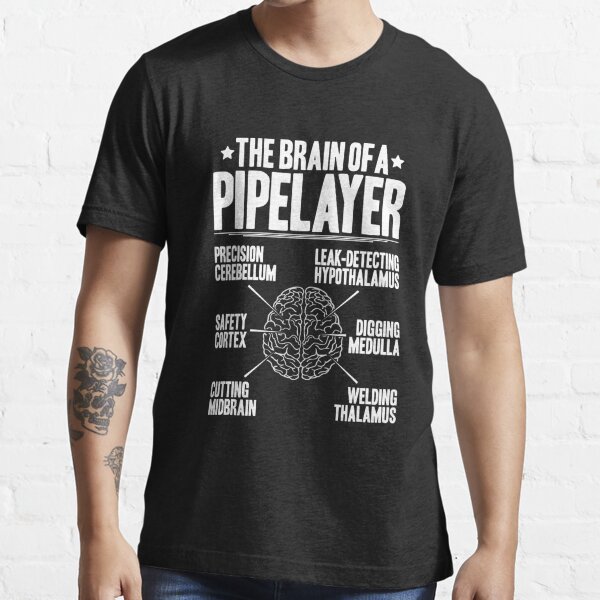The image is a color photograph showing a man from the neck down, standing in front of a white brick wall. He has tattoos on his right arm, including a prominent black tattoo of a flower atop a skull's head and a smaller heart tattoo below it. Additionally, there is another tattoo on the curve of his arm that appears to depict an explosion, though it's not entirely clear. He is wearing a gray t-shirt with a central design featuring a brain and various labeled sections around it. The text on the shirt reads "The Brain of a Pipe Layer," with labels such as "Precision Cerebellum," "Leak Detecting Hypothalamus," "Digging Medulla," "Welding Thalamus," "Cutting Midbrain," and "Safety Cortex" pointing to different parts of the brain illustration. At the bottom of the image, part of his blue jeans is visible.